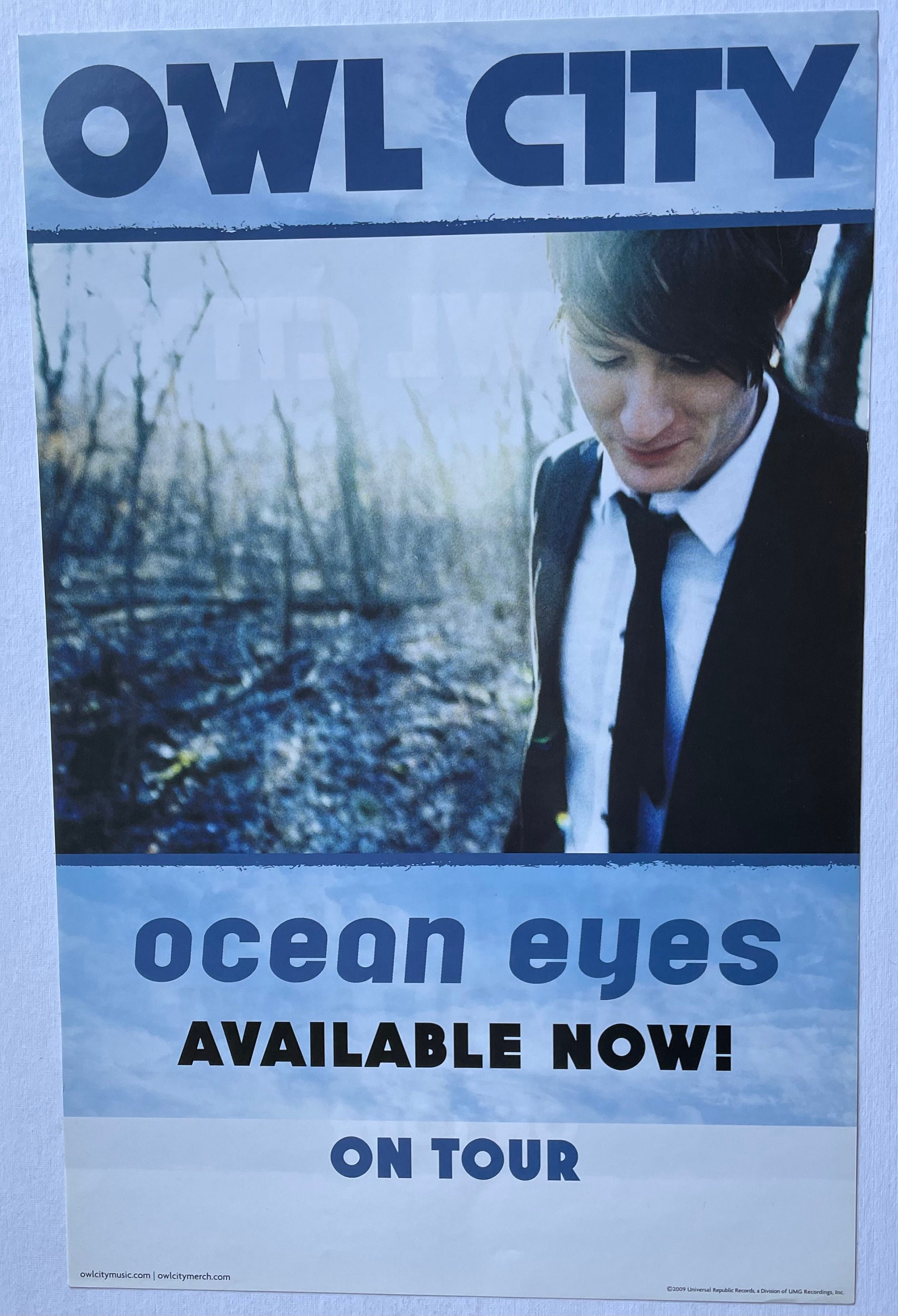The poster is an advertisement for a concert event or album release by the band Owl City. The top of the poster features the band’s name, "Owl City," in dark blue text against a blue background. Centrally placed is a photograph of the lead singer, who is positioned slightly to the right. He is depicted wearing a black suit jacket over a white button-up shirt and a black tie, with his dark brown hair swept to the left as he looks downwards. The backdrop appears to be an outdoor setting with blurred, leafless trees, indicating a fall or winter environment.

Below the photograph, in dark blue text, is the title "Ocean Eyes." Under this, in black text with an exclamation mark, it reads "Available Now!" followed by the words "On Tour" in blue text at the bottom. The poster has a white-bordered, cloud-like frame around the "Ocean Eyes" and "Available Now" text, enhancing the overall design. The bottom section also includes space presumably intended for tour date details. The border around the entire poster gives it a textured appearance, adding to its visual appeal.